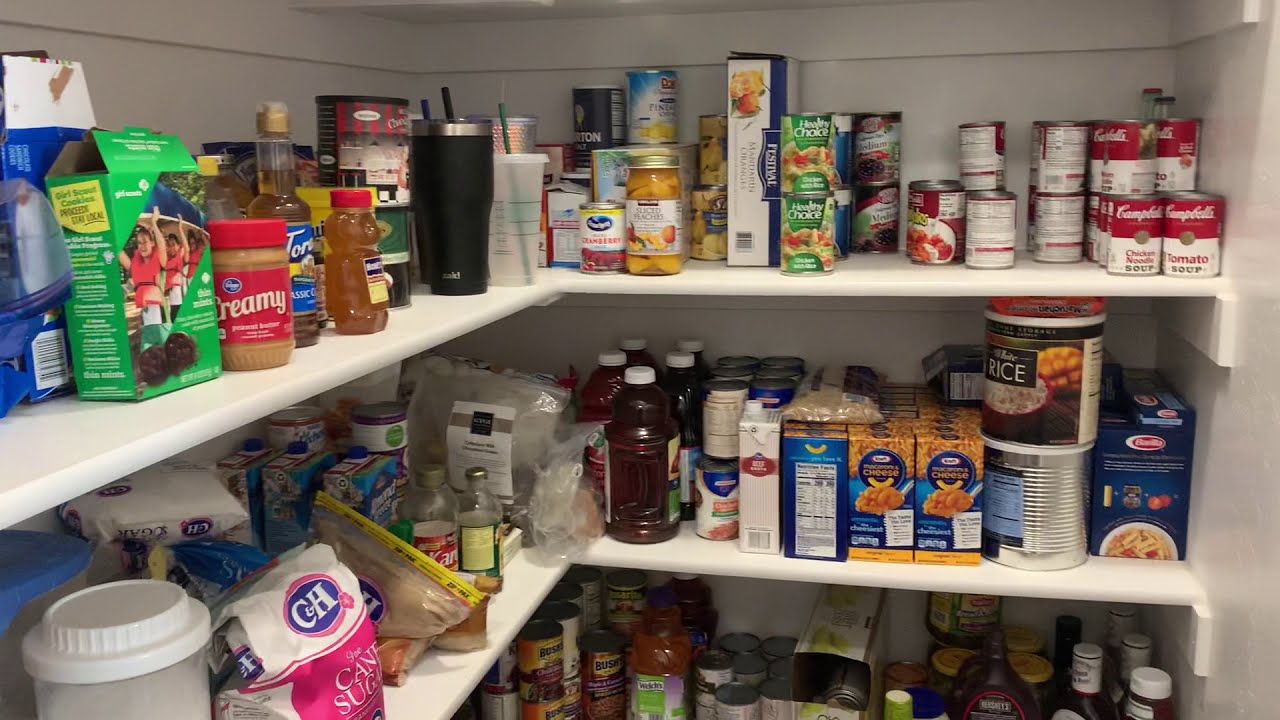This detailed image depicts a well-stocked pantry with six white, V-shaped shelves filled with a variety of food items. The top shelf features Girl Scout cookies, Kroger creamy peanut butter, Nesquik, honey, and several travel mugs. To the right, there's a collection of Campbell's soups, Healthy Choice soups, and cranberry jelly. Moving down to the next shelf, on the left, you can find a white and pink bag of cane sugar, brown sugar, and Karo syrup, along with Kraft macaroni and cheese, rice containers, and Barilla pasta. The bottom shelf, although a bit harder to see, contains barbecue sauce, Hershey's chocolate syrup, Welch's juice, and Bush's beans. The pantry's walls and shelves are painted white, creating a bright backdrop that highlights the colorful assortment of products.